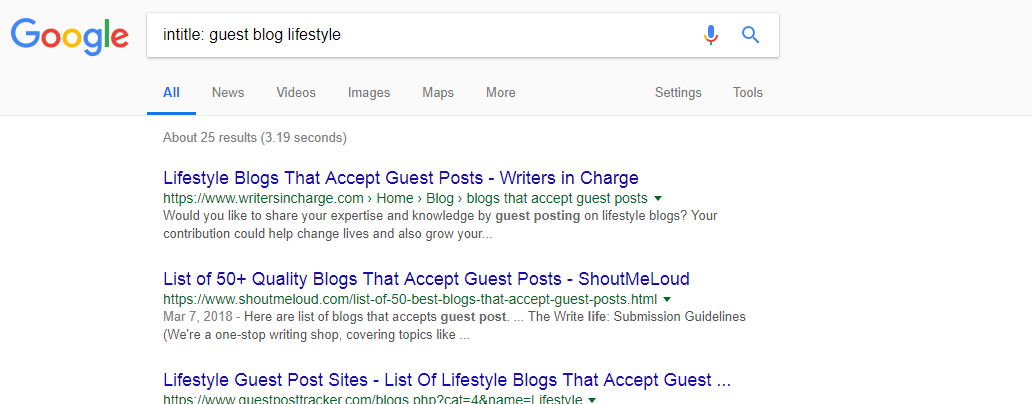This screenshot captures a Google search results page. The Google logo is prominently displayed in the top left corner, confirming the platform. At the top of the page, the search bar is positioned, featuring a microphone icon and a magnifying glass icon on the right side.

In the search bar, the user has input the query: `in title: "guest blog lifestyle"`. The user is currently viewing results under the "All" tab, which is highlighted in blue with a blue underline, signifying it as the active tab. Other available tabs include "News," "Videos," "Images," "Maps," "More," "Settings," and "Tools."

The search yielded approximately 25 results, displayed beneath the summary indicating the search duration of 3.19 seconds. The first few results listed include titles such as "Lifestyle Blogs That Accept Guest Posts - Writers In Charge," "A List of 50+ Quality Blogs that Accept Guest Posts - ShoutMeLoud," and "Lifestyle Guest Post Sites - List of Lifestyle Blogs That Accept Guest Posts."

This detailed view offers insight into the search query process and the initial search results for guest blogging opportunities in the lifestyle niche.